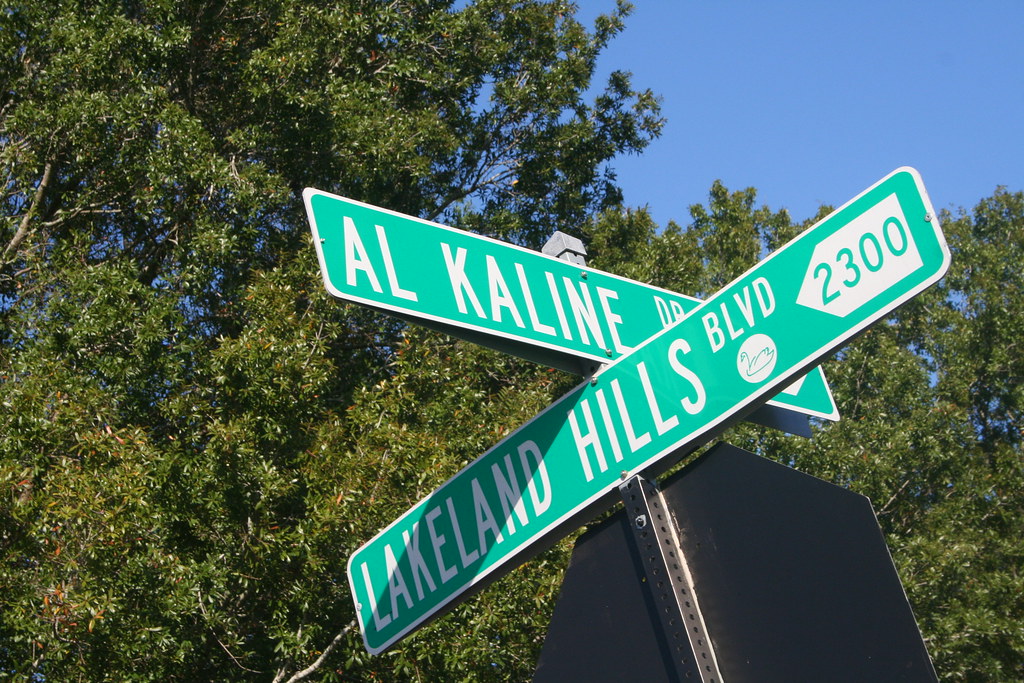In the image, a vibrant blue sky serves as a backdrop for lush green trees, their branches adorned with dense foliage. A prominent metal pole, marked with multiple holes, stands erect, supporting a stop sign with a visible gray backing on both sides. Adjacent to it is a green street sign reading "Lakeland Hills Boulevard," featuring a long, rectangular design with a white border and the number "2300" prominently displayed. Below the street signs, a house is partially visible, and nearby, an outdoor dryer can be seen. The scene combines elements of urban street signage with a suburban residential setting, all under a serene, clear sky.